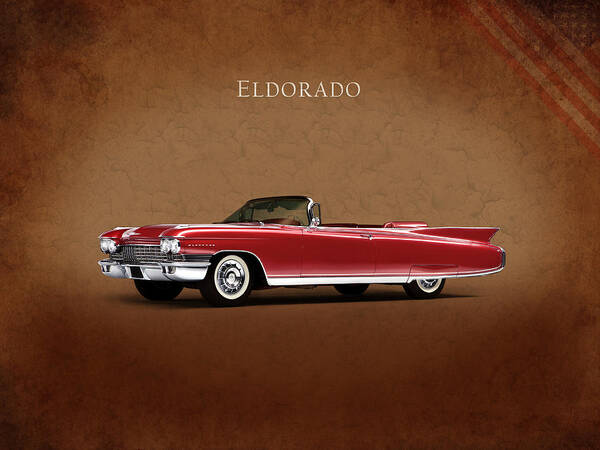This is a detailed advertisement poster for the Cadillac Eldorado, a classic red convertible from the 1950s or early 60s. The car, centrally positioned and horizontally elongated, features a cherry-red body with striking red fins at the back and a sloped windshield. It's equipped with four headlights, two on either side of the prominent chrome bumper. The Eldorado rides on black tires with white walls and showcases elegant silver trim. Above the car, the white text "Eldorado" is prominently displayed against a light brown background that transitions to a darker brown towards the corners. The backdrop also includes a blurred American flag in the top right corner, adding a patriotic touch to the sleek and aerodynamic design of this iconic vehicle.